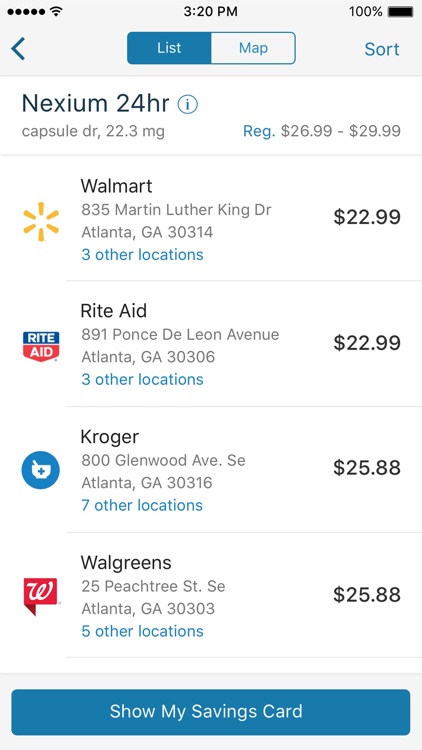Sure, here is the cleaned-up and detailed caption based on the voice description:

---

Screenshot of a phone screen showing a comparison of pharmacy prices for Nexium 24-Hour (22.3 mg capsules). The upper-left corner displays five black circular icons followed by three signal bars. Centered at the top, the time reads "3:20 p.m." To the right, the battery indicator shows 100% charge. Below this bar, a horizontal menu features a left-facing arrow on the left and two selectable tabs: a blue "List" tab with white text and a white "Map" tab outlined in blue with blue text. To the right of these tabs is a "Sort" option.

Below the menu, the page details the product "Nexium 24-hour," accompanied by a circled 'i' icon. The product specification reads: "Capsule DR, 22.3 mg," priced between $26.99 and $29.99. The screen then lists various pharmacies where the product can be purchased, including:

- **Walmart**: Icon with a yellow star, located at 835 Martin Luther King Drive, Atlanta, Georgia 30314, and three other locations, priced at $22.99.
- **Rite Aid**: Icon with the Rite Aid logo, located at 891 Ponce de Leon Avenue, Atlanta, Georgia 30306, and three other locations, priced at $22.99.
- **Kroger**: Icon with the Kroger logo, located at 800 Glenwood Avenue SE, Atlanta, Georgia 30316, and seven other locations, priced at $25.88.
- **Walgreens**: Icon with the Walgreens logo, located at 25 Peachtree Street SE, Atlanta, Georgia 30303, and five other locations, priced at $25.88.

The pharmacy names are in black font, the addresses in gray, and the "three other locations" text highlighted in blue. At the bottom of the screen, a blue box with white text reads "Show my savings card."

---

This detailed caption provides a comprehensive description of the screenshot's contents, including the layout, icons, text colors, and specific details about the product and its pricing at various pharmacies.